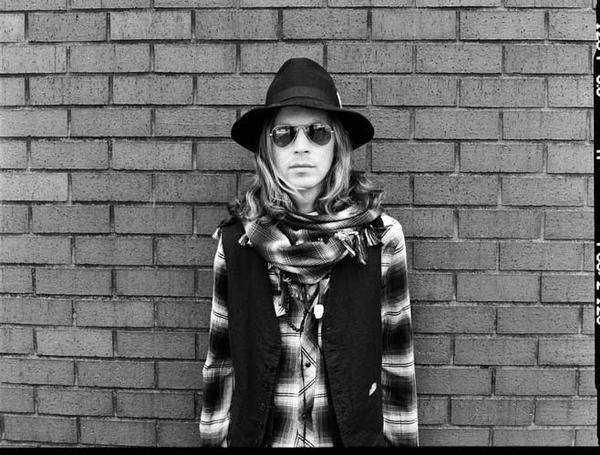In this black and white photograph, a man stands against a brick wall, looking directly at the camera with a straight, non-smiling expression. He wears a dark fedora-like hat that extends slightly above his head, resembling a cowboy hat. His shoulder-length hair, which appears to be darker at the roots and possibly blondish at the tips, cascades around a chunky black and white plaid scarf wrapped around his neck. He sports aviator sunglasses that reflect light on both sides. His attire includes a black and white plaid shirt layered beneath an open, dark vest, which features a right-side pocket with a small white piece of paper peeking out. The brick wall behind him varies in light and dark gray tones, serving as the sole background element, suggesting an outdoor setting though the monochrome palette offers no time-of-day indication. The overall appearance, enhanced by his attire and accessories, gives him a rockstar-like look.